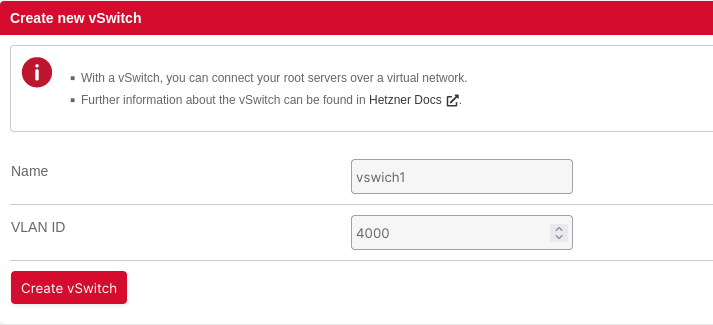This is a detailed caption for the given voice description:

---

This screenshot captures a website pop-up window for creating a new v-switch. The header at the top of the pop-up is in red, signaling urgency and importance. Below the header, there is an instructional message with a red eye icon. The message reads: "Create new v-switch: With a v-switch, you can connect to your root servers over a virtual network. Further information about the v-switch can be found in Hetzner Docs," with "Hetzner Docs" being a clickable, bolded link that redirects to the documentation.

Following the message, users are prompted to fill out two fields. The first field, labeled "Name," features an open text box pre-filled with "v-switch 1," where users can type in their desired name for the v-switch. The second field is labeled "VLAN ID," accompanied by a typable area and a drop-down box currently displaying "4000," allowing users to select or enter a VLAN ID number.

At the bottom of the pop-up window, there is a prominent red button labeled "Create v-switch," which draws attention to the action users need to take to finalize the creation of the v-switch. The overall color scheme of the pop-up is red and white, contributing to a clean, yet urgent and important, visual design.

---

This caption thoroughly describes the elements within the screenshot and conveys a clear understanding of the pop-up window's purpose and design.